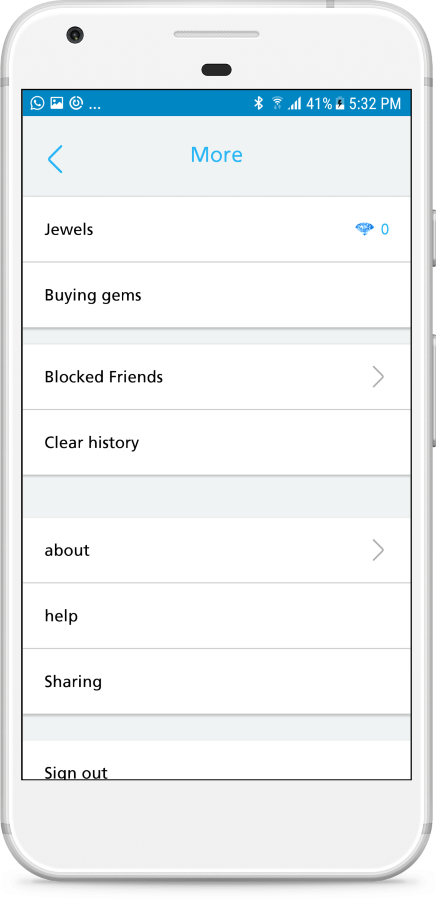The image features a mobile device showcasing a user interface with various elements. The device's upper part is white, featuring a small black hole on the left, likely a speaker or microphone. Centered at the top, there's a small oval shape below a longer, graded pattern slot.

At the top of the application screen, a blue strip is displayed. On the left side of this strip, a circular WhatsApp icon, resembling a white phone inside a speech bubble, is visible. Next to it, an image icon and a clock icon are positioned, followed by three vertical dots. On the right side of the blue strip, icons for Bluetooth, Wi-Fi, and data signal are displayed. The battery is at 41%, and the time is shown as 5:32 p.m.

Below this, a large gray strip spans the width of the screen, featuring an arrow pointing left with the word "More" in the center, all in light blue. 

The content is divided into sections by light gray lines. The first section, labeled "Jewels," is in bold black font, smaller than the "More" heading. To its right, a blue Wi-Fi signal icon and the number zero are displayed. The subsequent sections are titled "Buying Gems," "Blocked Friends," "Clear History," "About and Help," "Sharing," and "Sign Out." 

"Buying Gems," "Blocked Friends," "Clear History," "About and Help," "Sharing," and "Sign Out" have inconsistent capitalization compared to "Jewels." The "Blocked Friends" and "About" sections feature arrowheads pointing right, indicating navigable links. The background of these sections is a medium gray, similar to the "More" section.